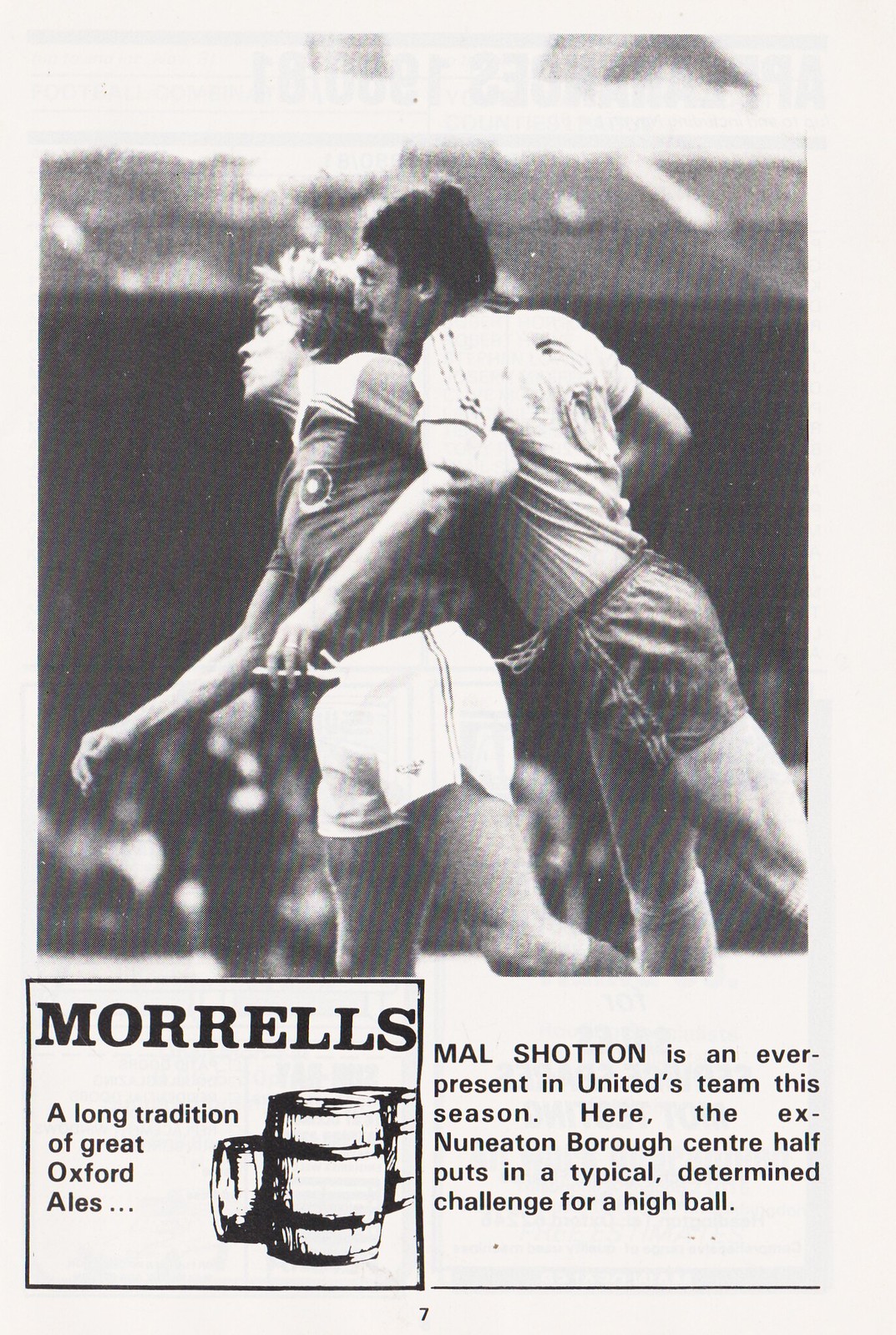The image is a magazine page featuring an advertisement. The top two-thirds showcases a black and white photograph of two soccer players in mid-collision as they challenge for a high ball. The player in darker shorts and a lighter jersey is seen jumping into the back of the other player, who is wearing white shorts and a darker jersey. Both have their eyes closed, with the front player displaying a pained expression and the back player an angry one. The bottom one-third of the page is divided into two sections. The left section features a black-bordered rectangle with the text "Morales, a long tradition of great Oxford ales" alongside an image of three wooden barrels. The right section contains a caption for the photograph, stating, "Mal Shotton is an ever-present in United's team this season. Here, the ex-Nunaton Borough centre half-foots in a typical determined challenge for a high ball." The page number "7" is also visible at the bottom center.